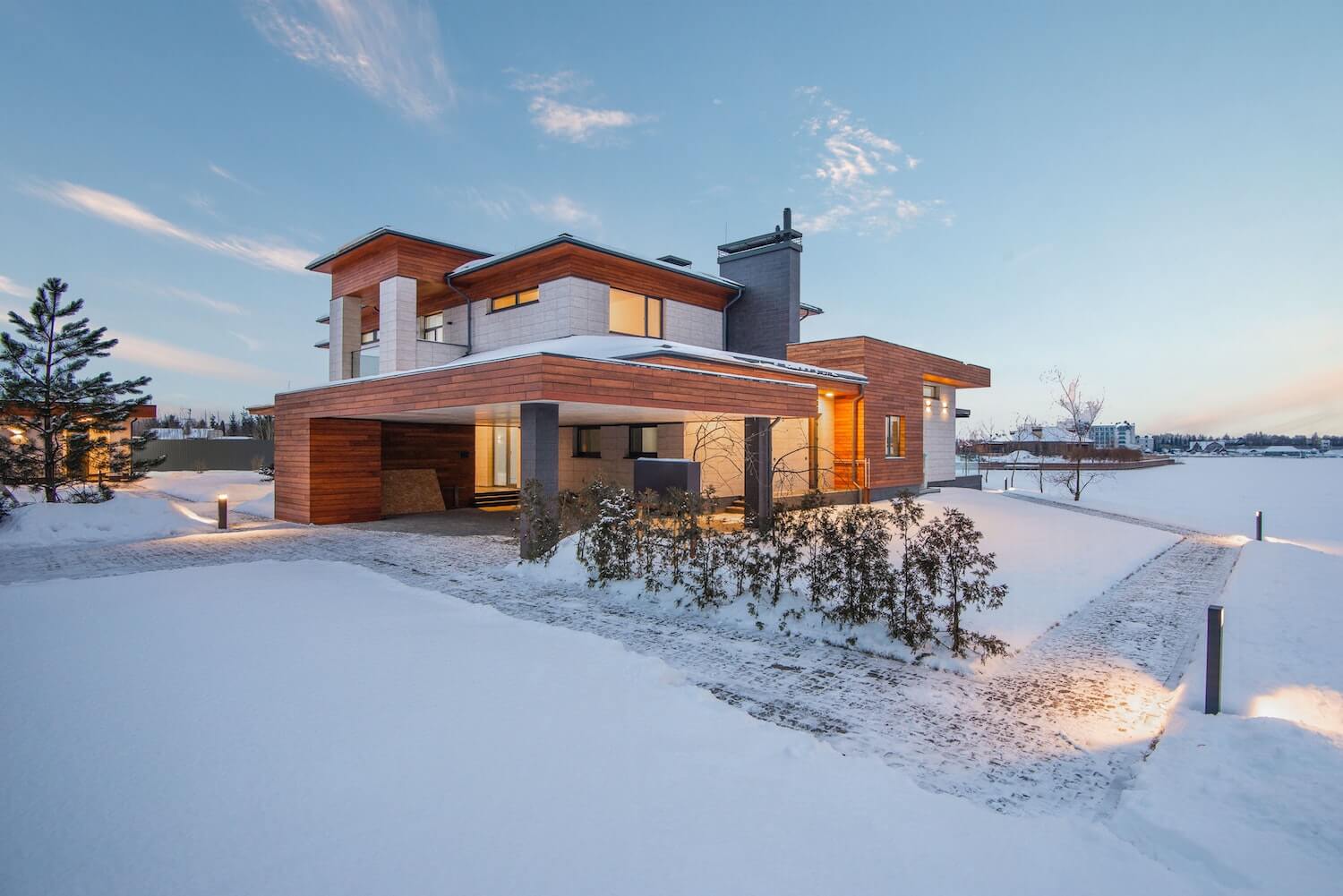In this image, we see a modern, Frank Lloyd Wright-style house set in a picturesque, snowy landscape. The house, composed of brown and white bricks, features flat planes and a notably broad, gray chimney extending from the roof. Gray, cubic columns are positioned under an overhang, serving as a carport area. The snow-covered ground envelops the space, with a shoveled pathway winding around the outer border of the property. Illuminated gray light stands add a warm glow to the scene. Flanking the house, snow-dusted pine trees and bushes contribute to the serene atmosphere. The sky, transitioning from light to darker blue as the day ends, is adorned with a few wispy clouds. In the background, additional buildings in brown and white and more trees can be seen, enhancing the sense of a quiet, snowy neighborhood.